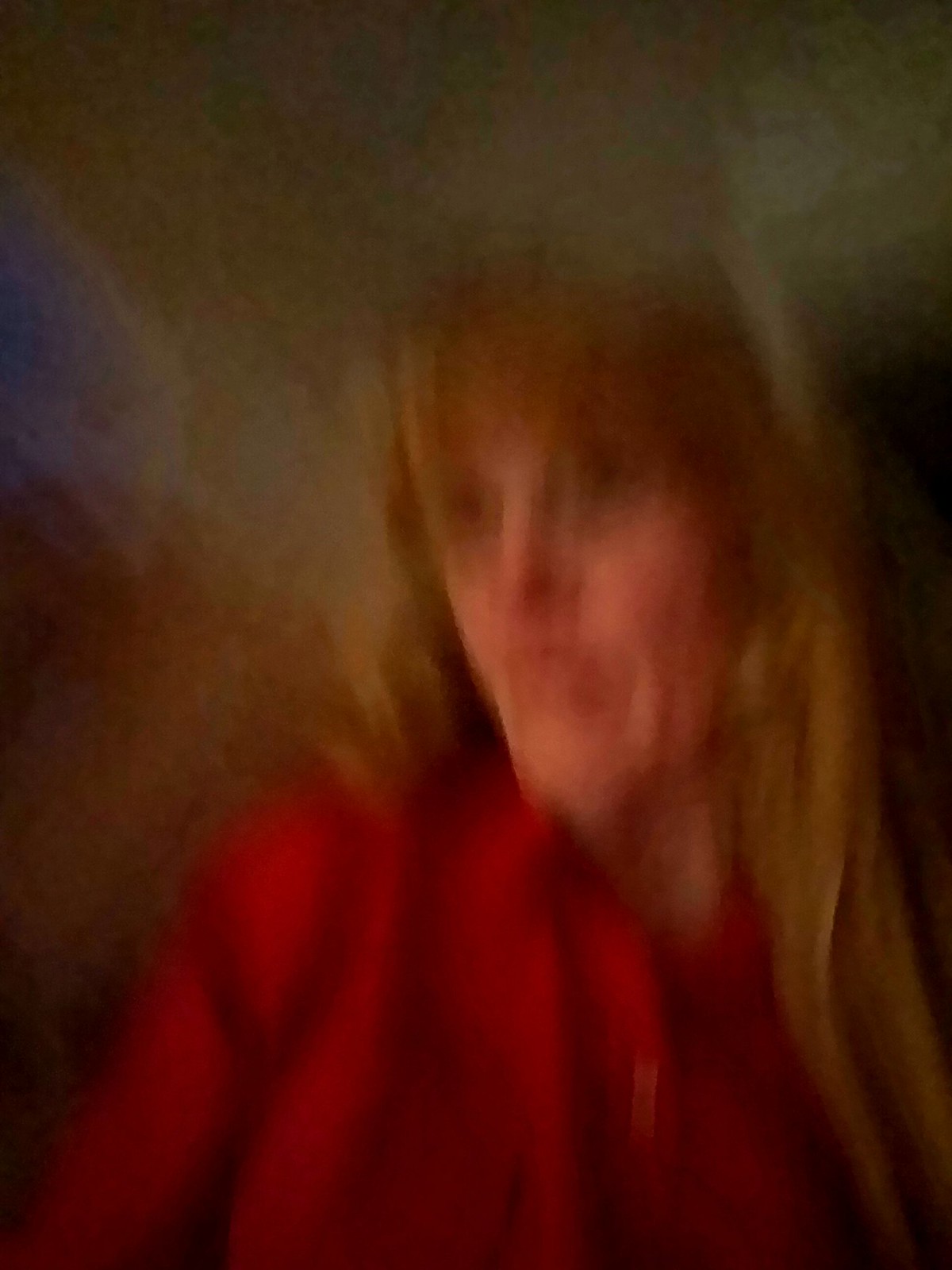A candid photograph of a woman accidentally capturing herself in a selfie. The blonde woman is seen wearing a red button-up shirt, standing out against the dimly-lit night backdrop. Her expression suggests the image was taken unexpectedly while she was in the process of looking at the camera. With fair complexion and subtle lighting, the overall ambiance of the photo hints at a casual, spontaneous moment.